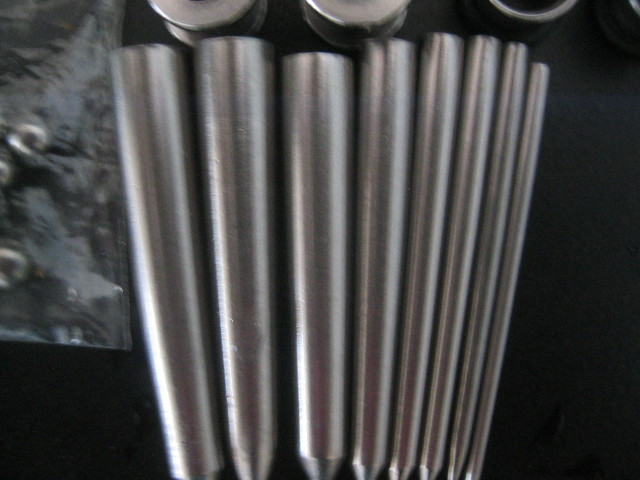The image depicts a blurry close-up photograph of several vertical, silvery metal cylinders, arranged in a fan-like formation against a black background. These cylinders, totaling about eight, vary in width, progressing from a thicker, wider cylinder on the far left to progressively thinner ones on the right. Each cylinder is capped with circular, silver metal knobs. The light source, possibly a flash, causes reflections on the metal surfaces, suggesting illumination from the viewer's perspective or behind them. Additionally, there are partial metal shapes, including cylinders and half-moon rounds, in the background that match the material of the standing cylinders. On the left side of the image, a blurry plastic object, potentially a bag, is visible. The intricate arrangement and reflections highlight the metallic texture and variation in cylinder sizes.